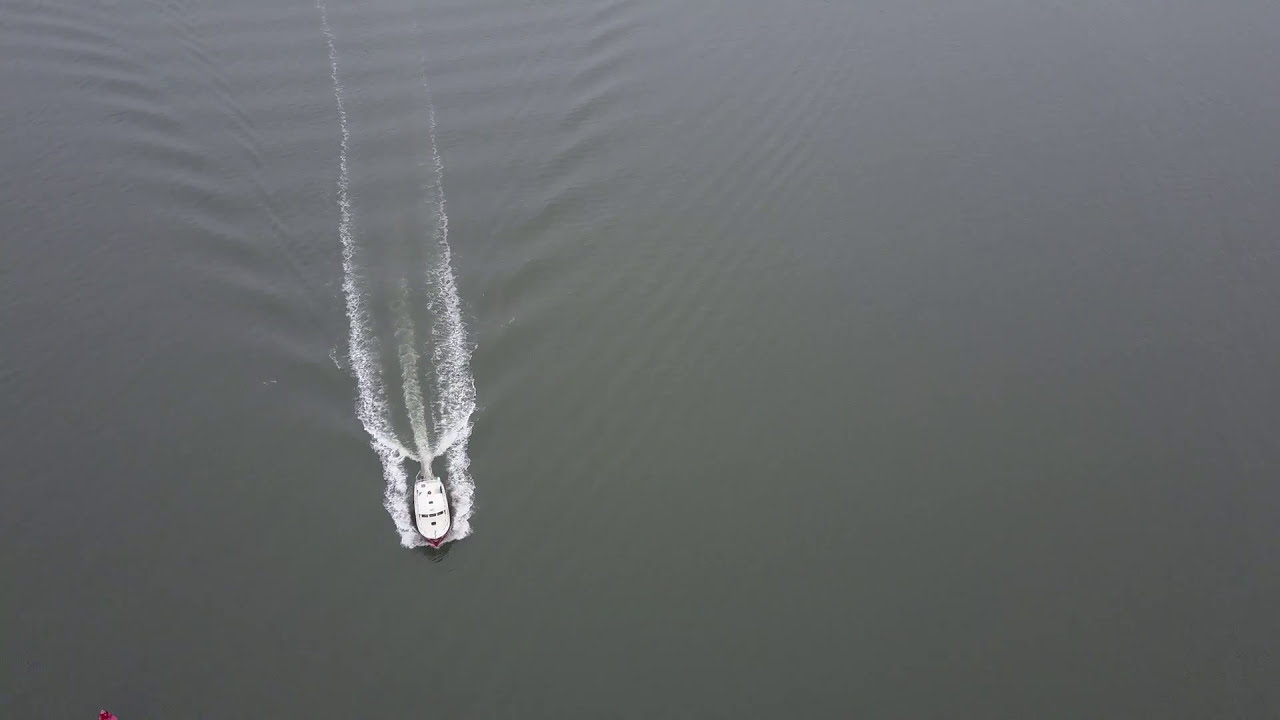This is an aerial photograph capturing a vast, seemingly deep, and still body of water, characterized by a consistent dark gray-green hue. The sole subject of the image is a small white boat, with a hint of red visible underneath, cutting through the water at a fast pace. Positioned about a third of the way from the left and roughly three-quarters down the landscape-oriented frame, the boat is traveling in a generally southward direction, around the 5:30 mark if visualized on a clock face. The boat's swift movement is evidenced by the pronounced V-shaped wake it leaves behind, with white-tipped ripples trailing off both sides and converging into a long, extended fishtail pattern. The image is devoid of any other elements, making the dynamic interaction between the boat and the tranquil water the focal point of this striking scene.